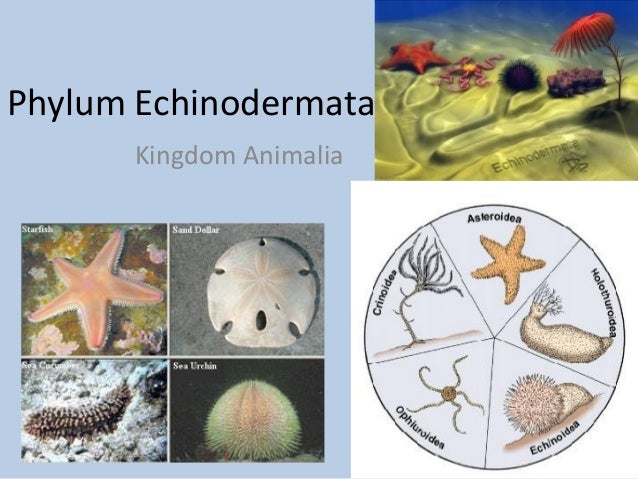The image features a detailed underwater scene filled with various marine animals, alongside their scientific classifications. Dominating the background is a blue ocean with a sandy bottom, populated by a red starfish, what appears to be an octopus, and a black sea urchin. In the bottom left corner, there's a four-part inset showing actual photographs of marine creatures: a starfish in the ocean's depths (upper left), a tan and white sand dollar (upper right), a sea cucumber (bottom left), and a green sea urchin (bottom right). Additionally, the image includes a pie chart on the bottom right, presenting marine animals in each slice. Text overlays indicate the categories "Phylum Echinodermata" and "Kingdom Animalia" in black and gray lettering, respectively, with labels for each animal. There are also scientific names displayed next to the images, adding to the educational aspect. The color palette includes shades of blue, red, tan, white, and black, blending real and drawn visuals to create an illustrative and informative scene likely meant for educational use.